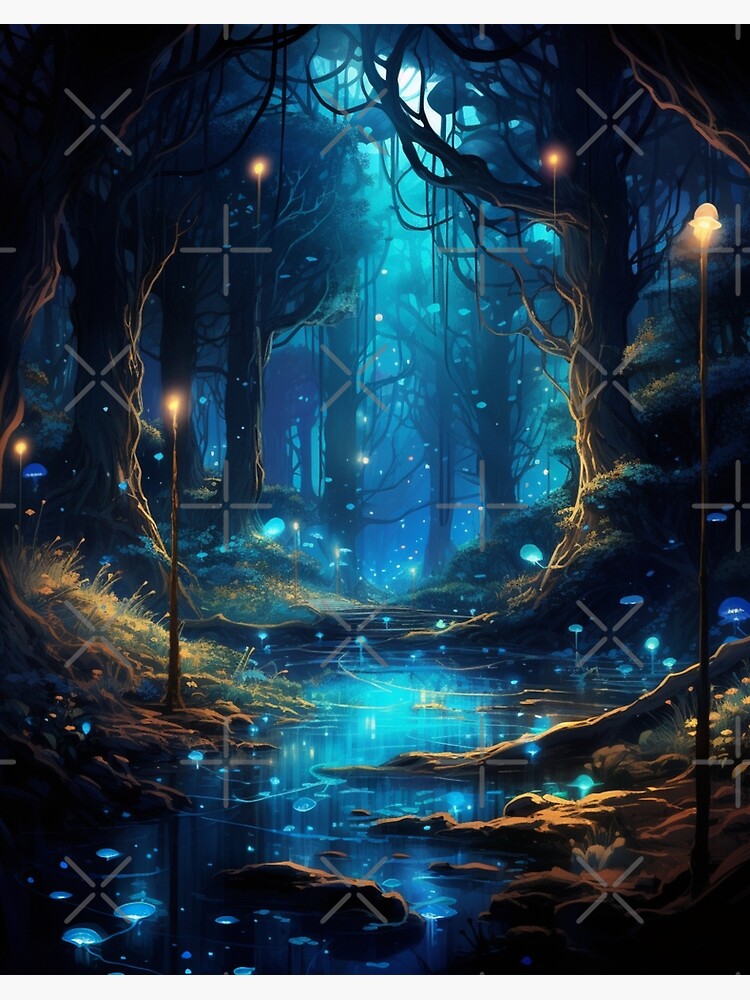The image is a vibrant, animated drawing depicting a surreal forest scene. A brilliant light blue stream of water winds its way from the lower center toward the upper background, cutting through a dense array of brown trees. Some branches reach into the water, extending to the right and left centers of the drawing. Scattered across both sides of the picture are white Xs or crosses, adding a mystical element to the scene. Larger trees with thick trunks dominate the background, while smaller trees and intertwining shrubs fill the foreground. The overall color palette includes bright neon blue, navy blue, black, green, and brown, enhanced by glowing illuminated lights ranging from blue to yellow and orange. The top of the image fades into darkness, suggesting dusk. Grass and flowers grow in the bottom right corner, with patches of brown mud and dirt visible, punctuated by blue floating bubbles. The entire setting is bathed in natural light, making the vivid details and colors stand out clearly.